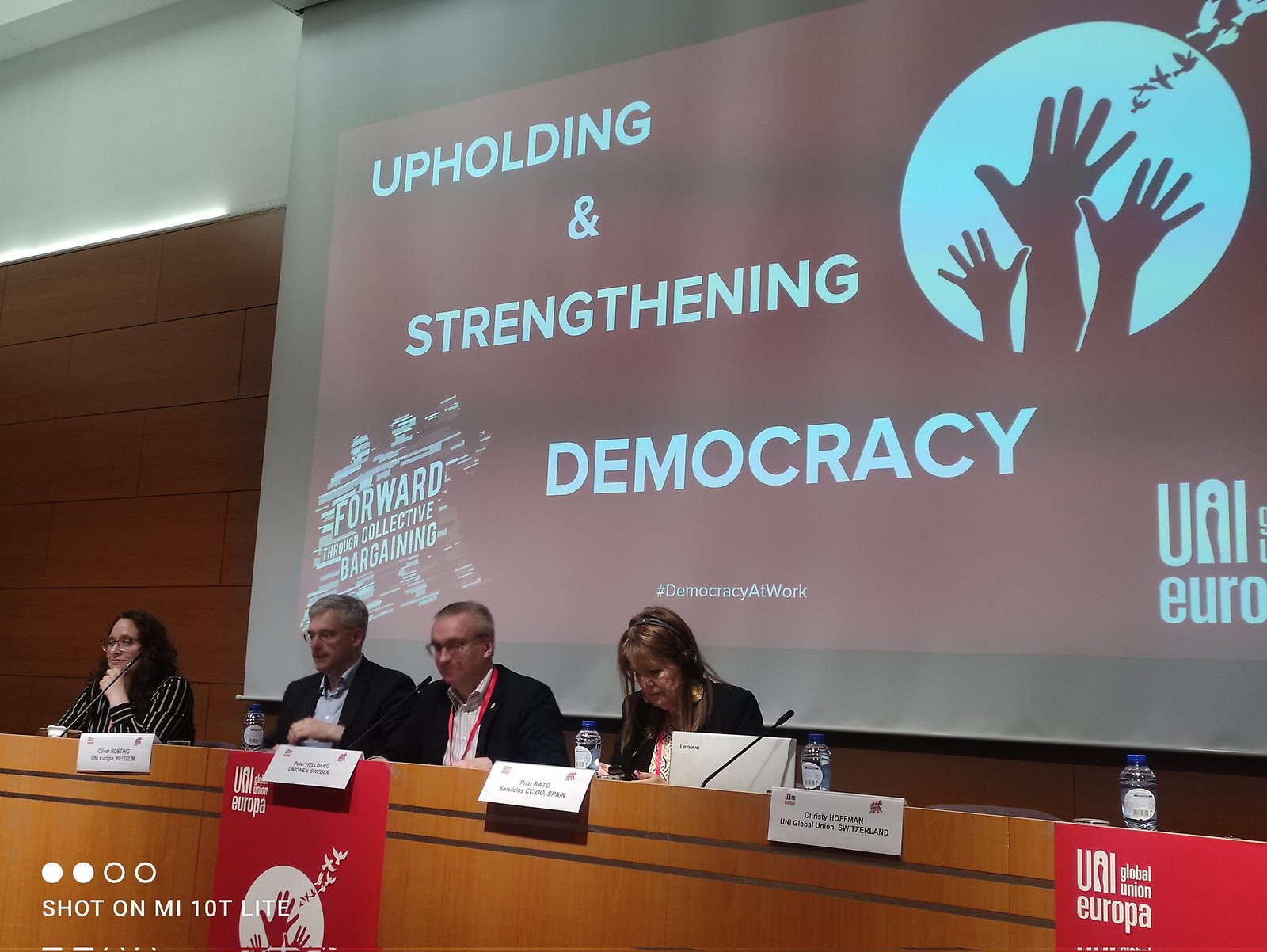The color photograph in landscape orientation depicts a panel of four people speaking at an event, seated behind a wooden table with microphones and name placards. The podium, set against a backdrop, features a combination of clean white and wood-paneled walls adorned with large rectangular wooden squares. Dominating the right-hand side of the image is a large screen with a red background, displaying the message "Upholding and Strengthening Democracy" in bold white letters. The upper right corner of this screen shows a white circle with the shadow of three hands inside it. Additionally, red banners matching the screen's circle and hand motif flank the wooden wall behind the panel. From left to right, the panelists include a woman with long dark hair wearing a black and white striped shirt, a man in a dark blazer with a light shirt, another man in a dark blazer with a pink shirt and a red hang tag, and lastly, a woman with long dark hair dressed in a dark blouse, who appears to be examining something on the desk. The realistic, photographic image captures the formality and focus of the event, emphasizing the theme and the involvement of the speakers.